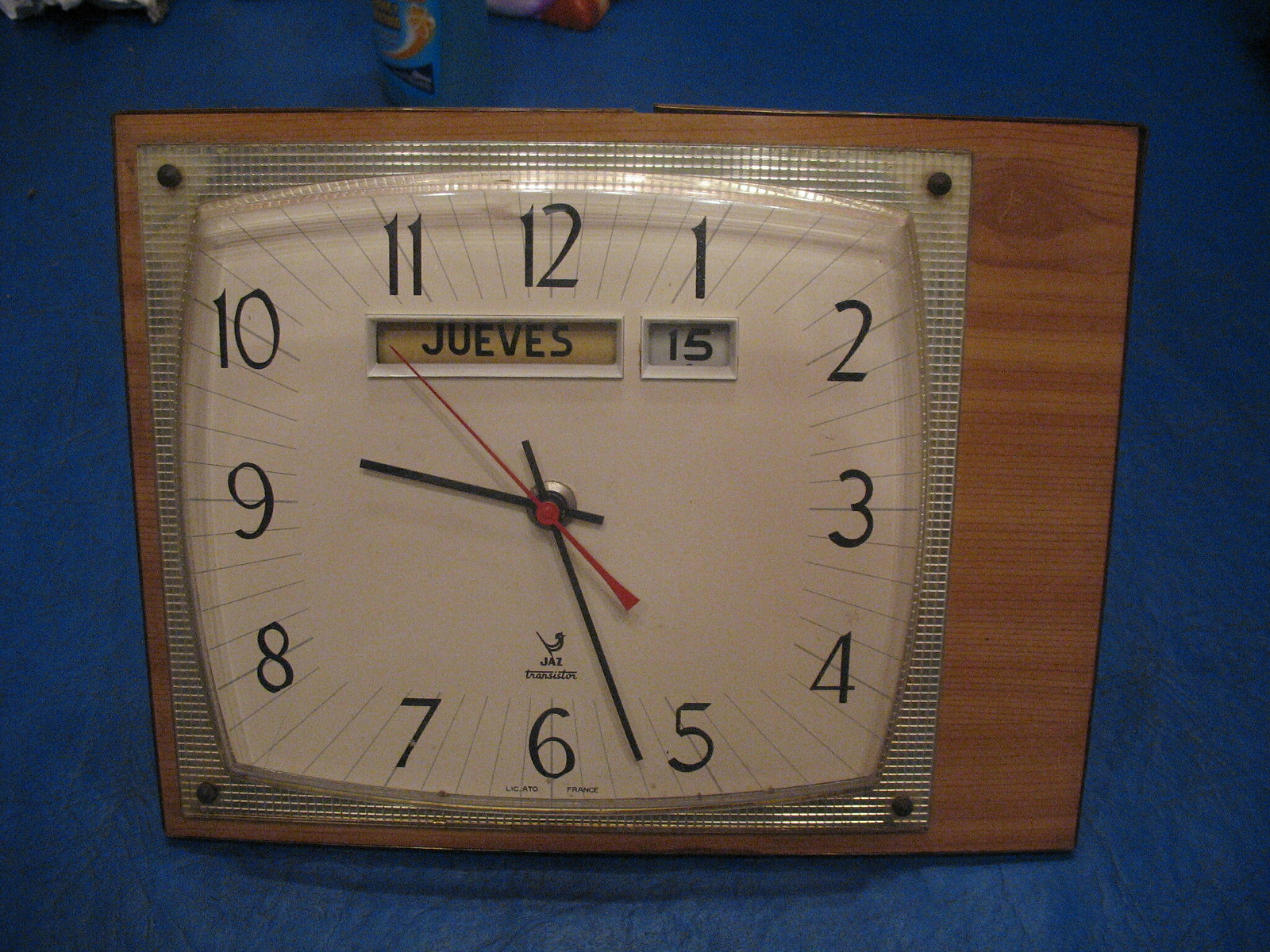The image features a richly colored royal blue wall with subtle light grey marbling streaks that add a textured elegance to the background. Prominently mounted on this wall is a wooden board that exudes a warm, natural tone. Affixed to the wooden board is a distinctive square clock with a mesh-like design on its face, offering a blend of traditional and contemporary aesthetics. The clock itself is highly detailed, featuring all twelve numbers in a clear and readable font, along with precise minute markers around its circumference. 

Noteworthy details include a small bird emblem perched on the front of the clock, adding a charming and whimsical touch. The clock is equipped with hour, minute, and second hands, ensuring accurate timekeeping. An important detail on the clock's face is the inscription "Jouves 15," indicating the current date. The time displayed is approximately 9:27. The combination of the textured blue wall, the wooden board, and the uniquely designed clock creates a visually striking and meticulously detailed focal point.